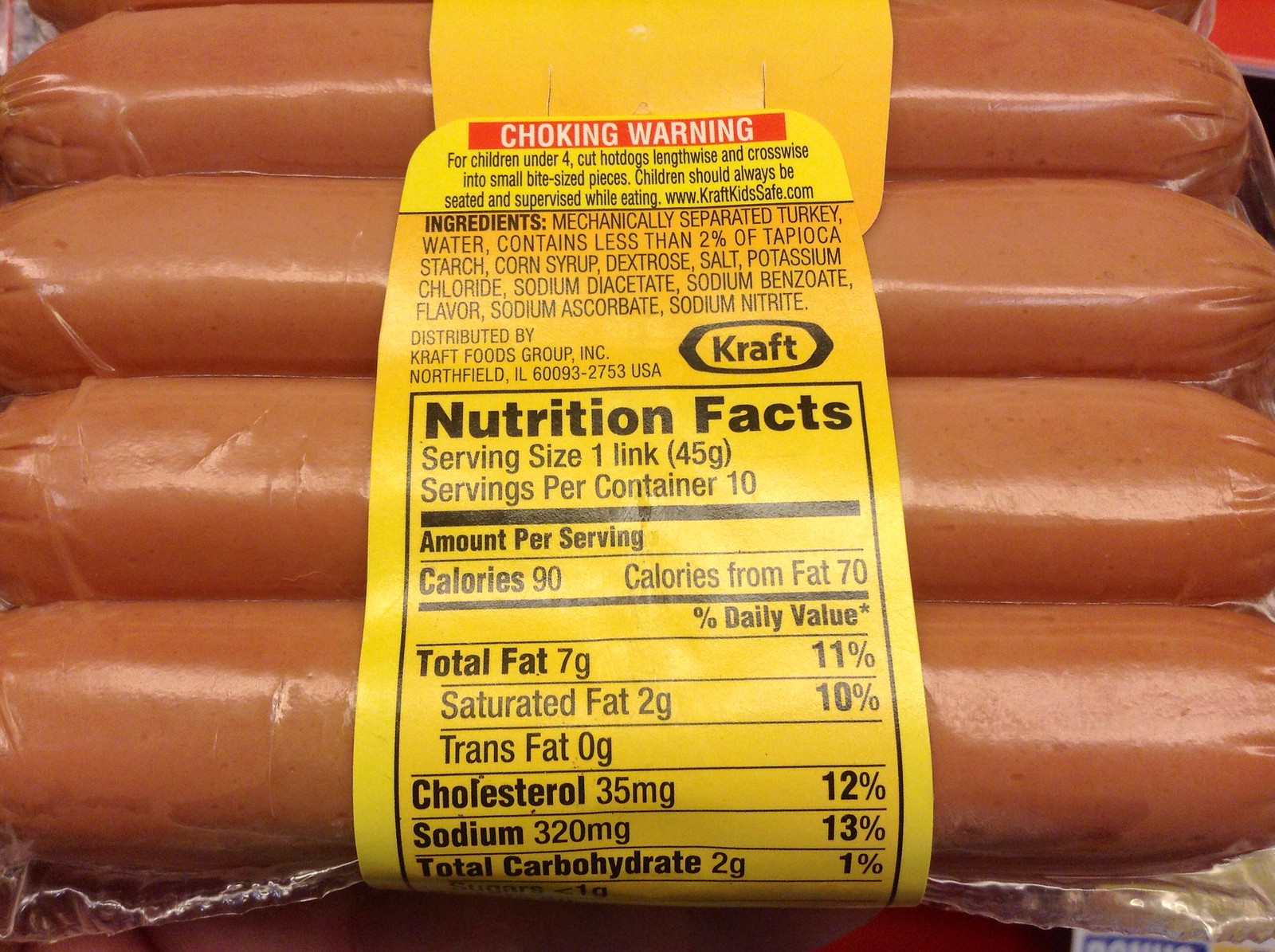This photograph captures a close-up of Kraft hot dogs taken from the bottom side up, prominently displaying the yellow nutrition label. The hot dogs are encased in a clear cellophane package, revealing their pale pinkish hue. The image clearly shows four elongated hot dogs, with a suggestion of an additional row beneath them. The nutrition label is the focal point of the image, wrapped around the package. A notable feature at the top of the label is an orange banner with a white text warning about the choking hazard for children under four years old. The banner advises cutting the hot dogs lengthwise and crosswise into small, bite-sized pieces and emphasizes the importance of children being seated and supervised while eating. The nutrition facts listed indicate that the total fat content is seven grams, with the package containing ten servings.